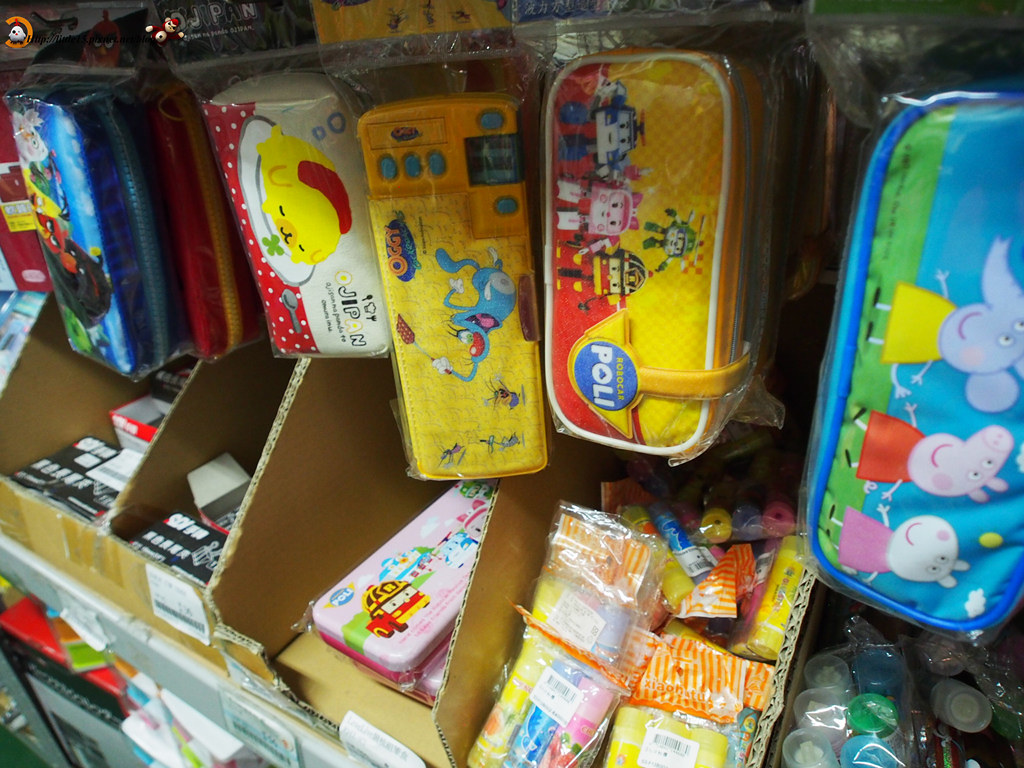This image depicts a section of a retail store, likely within a children's or baby aisle, featuring an organized display of soft-sided, zippered pencil cases. These pencil cases are hung neatly from pegs, each encased in plastic. On the far right, there is a blue pencil case adorned with characters from the popular children's show "Peppa Pig." Next to it, a yellow pencil case displays a robot figure. Other pencil cases feature various designs, including a cat holding a spatula and an animated dog, although some characters remain unidentified. Below these hanging items, a shelf showcases partially cut-away cardboard cartons revealing an assortment of colorful objects, some of which appear to be glue sticks. Another lower shelf contains large, colorful boxes, though the text on these boxes is not decipherable in this image. The overall scene suggests a vibrant, well-stocked area catering to children's stationery and small toys.